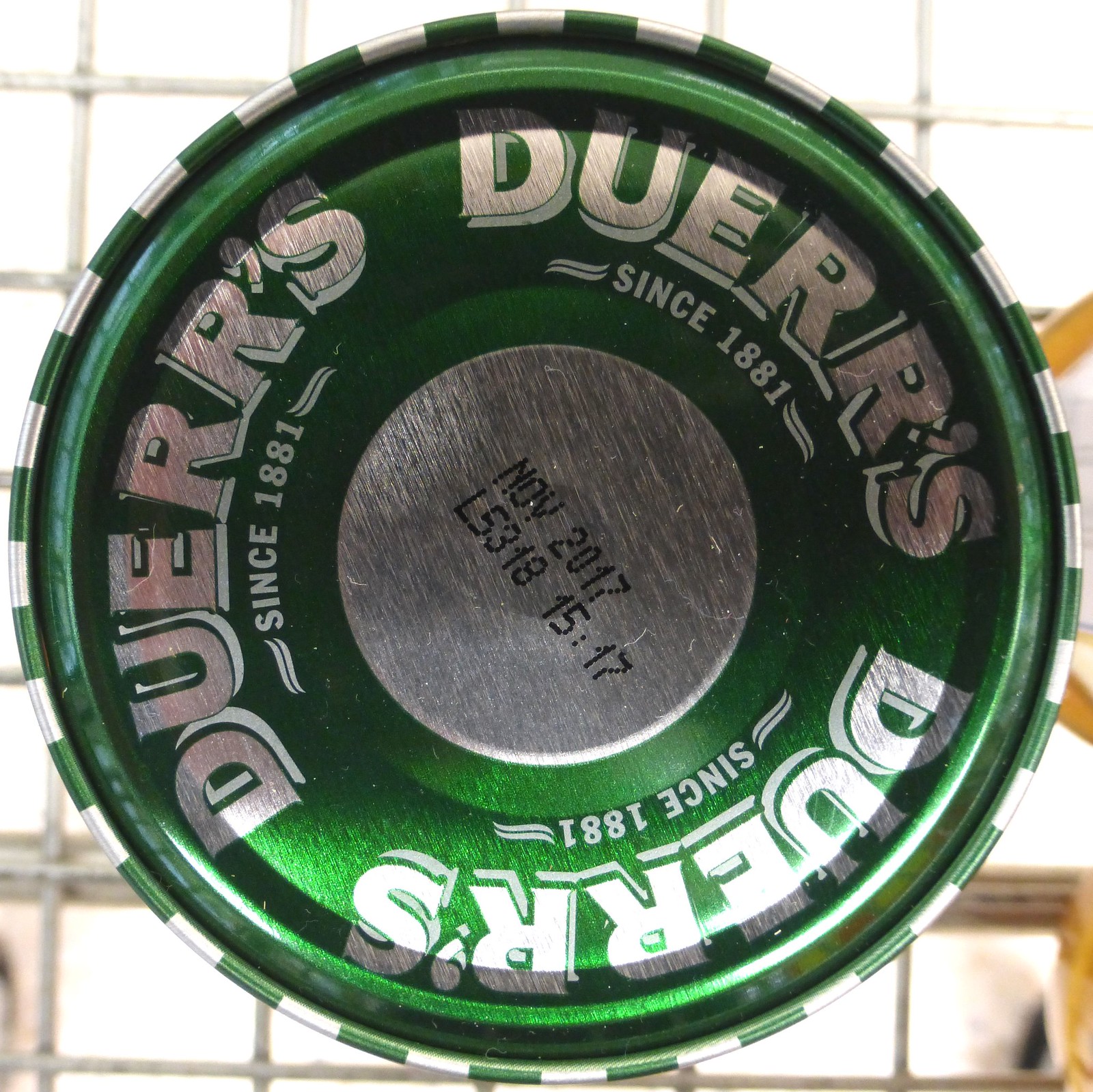The image depicts a green and white striped bottle cap resembling a poker chip, adorned with intricate details. At the center of the cap lies a silver, pop-up seal indicating whether the bottle has been unsealed. Surrounding this seal, in black text, is a date reading "November 2017, 15:17, 3:17 p.m.," though it is unclear whether this marks the production or expiration date. Encircling the middle of the cap, the name "Duerr's" is prominently repeated three times in shiny silver letters, a nod to the company's long history since 1881.